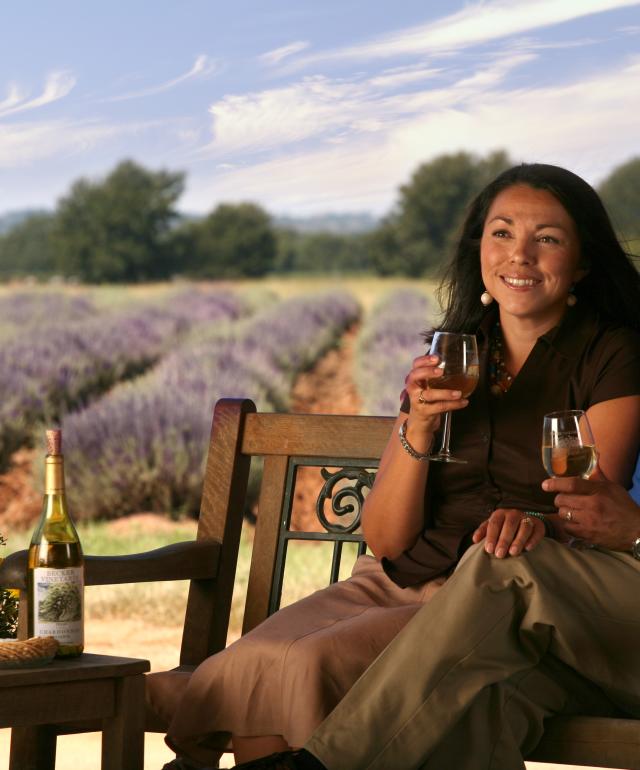The digital photograph captures a joyful woman seated on a dark wood bench with an ornate black metal design on the back, set outdoors against a picturesque backdrop of rows of tall, purple vineyard plants with dirt paths between them and trees in the distance. She is dressed in a black shirt and a tan skirt and wears a silver wristwatch. The woman is smiling warmly, holding a half-full glass of white wine in her right hand, poised to take a sip. Her left hand rests on the knee of a companion, whose partial presence is indicated by visible beige slacks. The companion also holds a half-filled wine glass. In the bottom left corner, a table displays a bottle of wine from Becker Vineyard, notable for its elegant gold-colored top, complementing the sophisticated ambiance of the scene. The overall color palette features rich greens, purples, dark reds, and browns, enhancing the visual appeal of this serene vineyard setting.